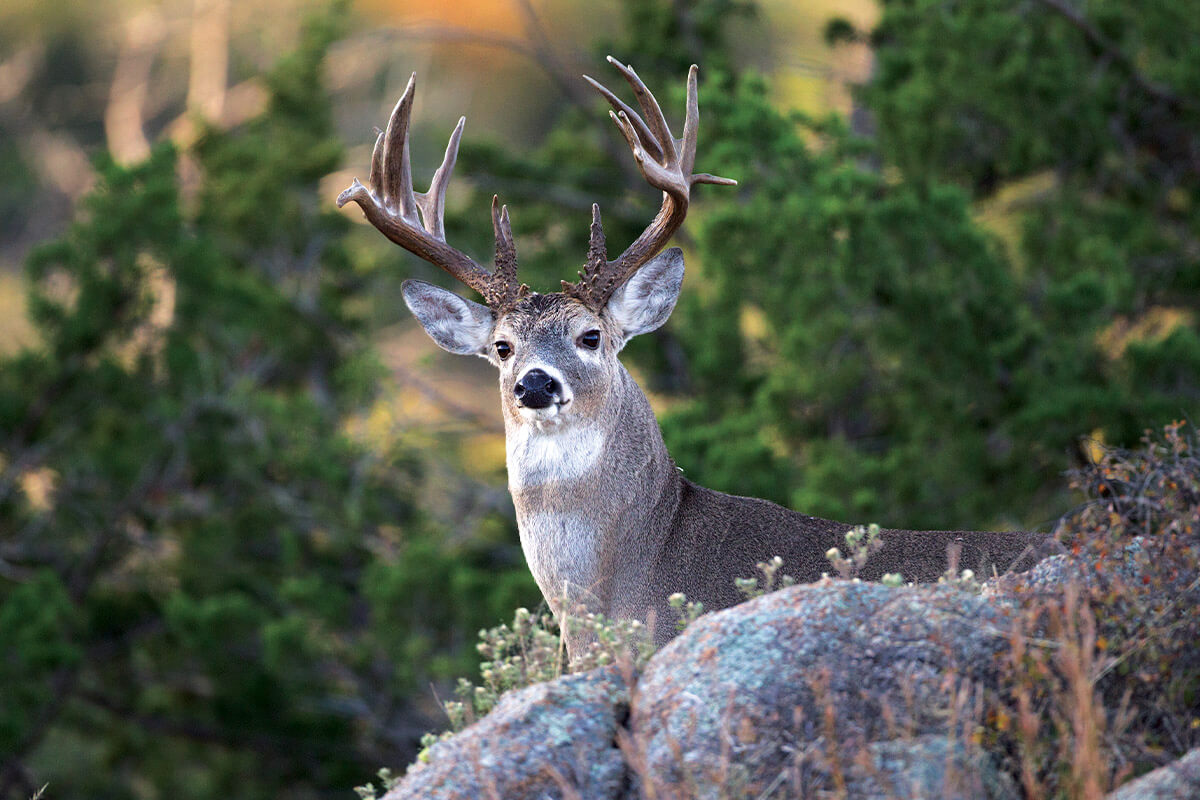In the photograph, a vigilant white-tailed deer stands partially obscured behind large, gray boulders. Nestled among the rocks, hints of reddish-orange and green grasses with yellow tips add a splash of color. The deer's sturdy, sharp brown antlers, showcasing four to five smaller spikes, arc gracefully with some curving toward each other. Its body faces slightly to the left, though mostly hidden, while the head and upper torso dominate the center of the image as the deer gazes directly at the camera with black eyes and a black nose. Its ears are perked up, revealing white interiors, and its brown coat contrasts with a lighter neck and a whitish chin. Behind the deer, a lush forest setting is evident, with the background displaying blurry green trees and touches of yellow and orange foliage, suggesting the picture was taken in broad daylight within a vibrant jungle or forest environment.